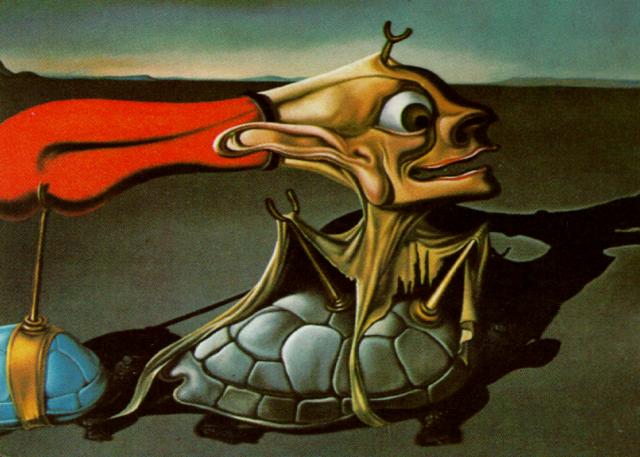In this abstract painting reminiscent of Salvador Dali's surrealist style, the focal point is a grotesque, skinned human face wearing a red hat. This distorted face, with wide, startled eyes and an elongated mouth, is mounted on metallic rods attached to a dark brown turtle with a shiny grey shell. The turtle's two right legs and head are visible as it moves toward the right. Supporting the rear of the outstretched head is another turtle, smaller in size, with a blue shell and a bronze-like rod stemming from its back. The background features a desert-like landscape with hazy, distant mountains beneath a sky that transitions from dark grey at the top to white near the horizon. The ground beneath the turtles and the surreal creature is a uniform dark grey, casting faint shadows and emphasizing the eerie, dreamlike atmosphere of the scene.